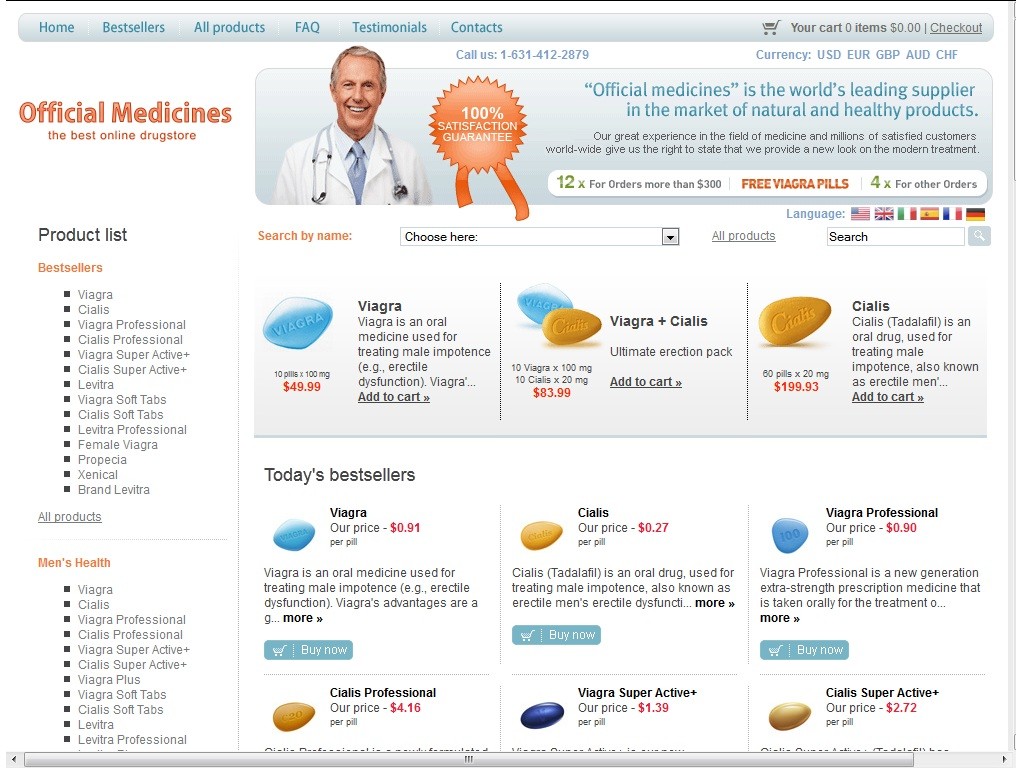This image from Official Medicines, an acclaimed online drugstore, depicts a professional figure that appears to be a doctor. The man is outfitted in a pristine white lab coat and a light blue tie, with a stethoscope draped around his neck, symbolizing his medical expertise. Positioned beside him is a ribbon proclaiming a "100% Satisfaction Guarantee."

Above the doctor, the website's navigation bar, set against a gray background, lists categories such as Home, Best Sellers, All Products, FAQ, Testimonials, and Contacts. On the left sidebar, a detailed product list includes items like Viagra, Viagra Plus Cialis, Cialis, Today's Best Sellers, Viagra Professional, Cialis Professional, Viagra Super Active, and Cialis Super Active.

The banner above highlights a promotional offer: "12 free Viagra pills for orders over $300, 4 free pills for other orders." The tagline below affirms, "Official Medicines is the world's leading supplier in the market of natural and healthy products," emphasizing their vast experience and millions of satisfied customers as proof of their authority and innovation in modern medical treatment. The overall background of the website remains predominantly white, with a subtle light halo effect around the doctor, drawing focus to him.